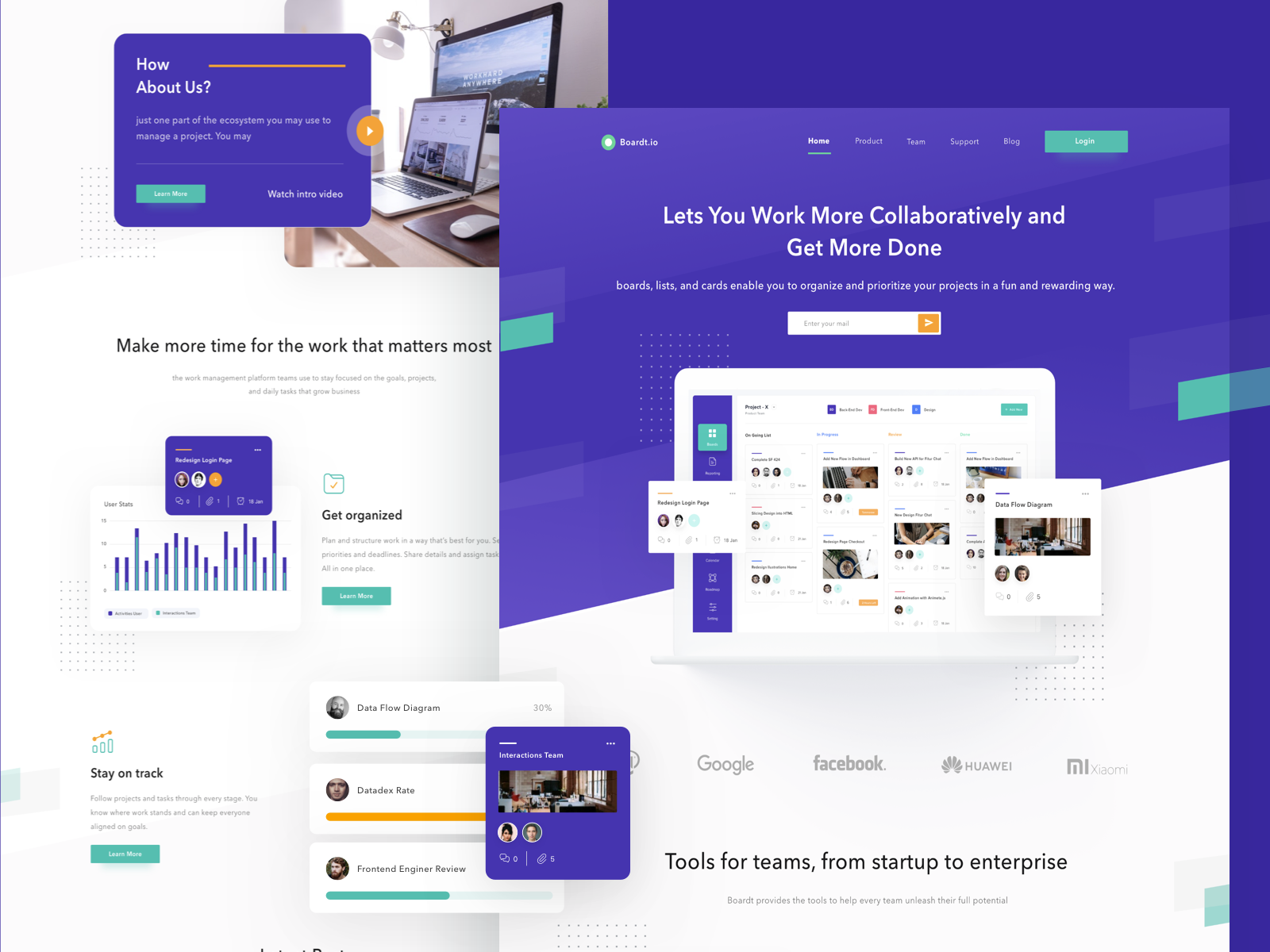This image depicts a comprehensive and collaborative webpage interface designed for teamwork and project management. At the top left, there is a background screen with a navigation menu on the left-hand side that includes "How" and "About Us" sections, set in white text against an indigo background. An orange horizontal line sits at the top of the page. Below the main navigation, lighter text reads, "This is just one part of the ecosystem you may use to manage a project." To the right of this text is an orange play button.

The main section of the page features a prominent slogan, "Make more time for what matters most," displayed in black text over a white background with a gray gradient on the right. Below this, there is a widget displaying bar graphs titled "Get Organized," with a teal hyperlink box below it labeled "Data Fixer Program." There are two more options under this section, with the top option showing a one-fourth full teal progress bar partially obscured by an indigo box to the right.

On the right side of the image, a larger screen showcases what appears to be the main webpage, possibly labeled "Breach IO." At the top of this screen are navigation labels in white text for "Home," "Product," "Team," "Support," and "Blogging," with a teal login button in white text to the right. The top part of this section is set against an indigo background with another message below it reading, "Let you work more collaboratively and get more done." Further down, it states, "Boards, lists, and cards enable you to organize and prioritize your products and have fun and rewarding experiences."

A search bar with an orange search button is positioned beneath this section, followed by another image resembling the same webpage. Concluding the page are logos of companies such as Google and Facebook, with a caption that reads, "Tools for teams from startup to enterprise."